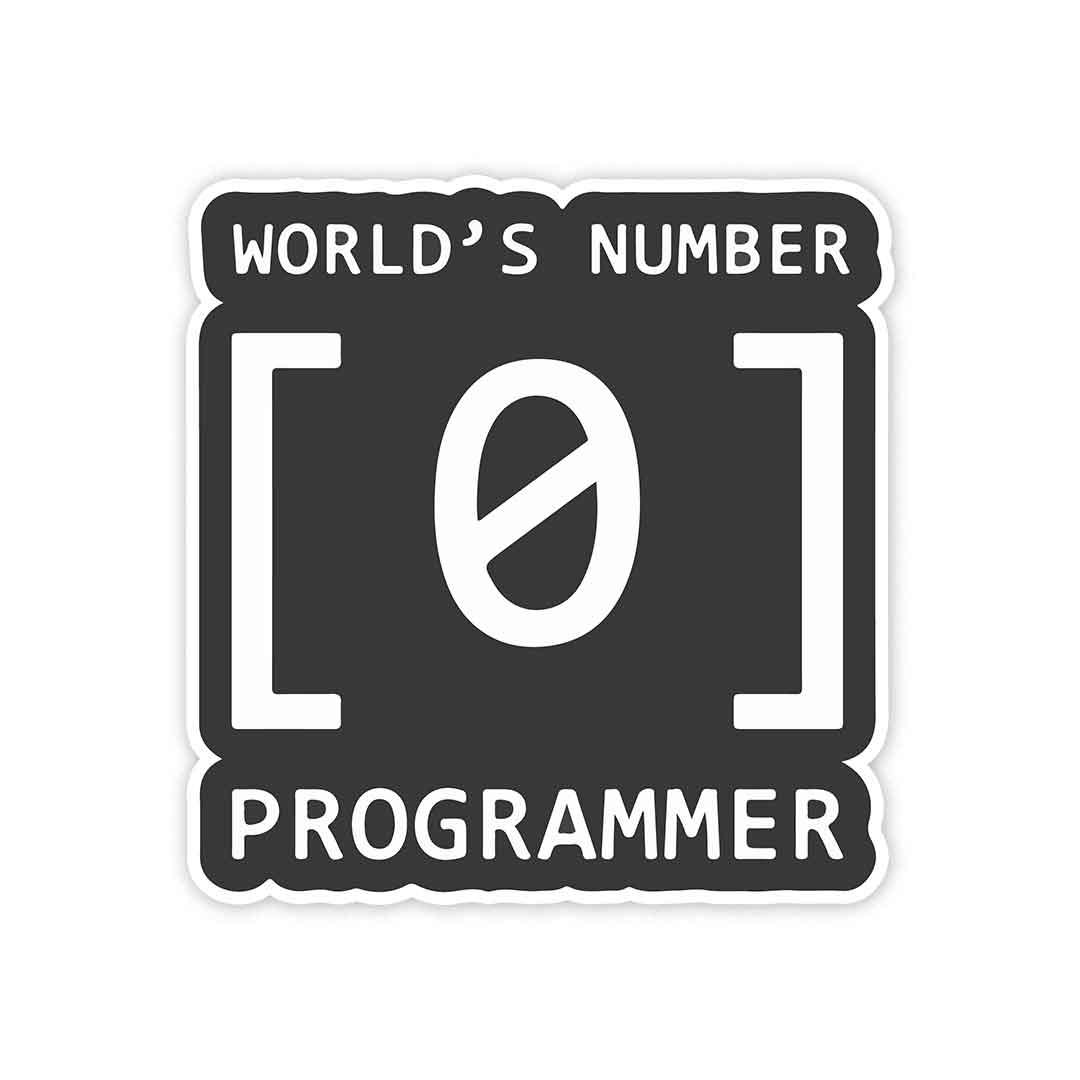The image is a dark gray advertisement bordered with a white trim that contours around the text. At the top, "WORLD'S NUMBER" is written in large white uppercase letters. Dominating the center of the image is an even larger set of white characters: a zero enclosed in square brackets [0], clearly marked with a stroke through the zero to distinguish it from an 'O'. At the bottom, the word "PROGRAMMER" is written in white uppercase letters. The text is arranged in a way that the border ripples slightly around the letters, creating a dynamic visual effect. This black and white sign humorously suggests that the programmer is ranked "world's number zero," likely as a playful commentary or a customizable graphic for various purposes.